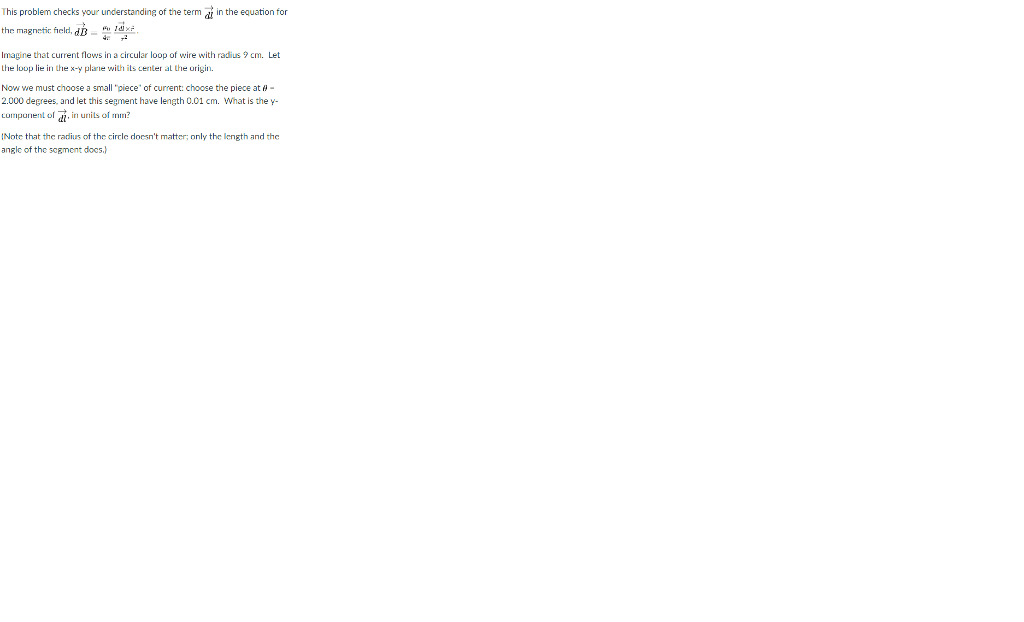This image features a very small square section of text that appears to be an excerpt from a mathematics or physics problem. The text is difficult to read due to its minuscule size, even when zoomed in. From what can be discerned, the problem checks the understanding of certain terminologies and includes equations related to the magnetic field.

The readable part of the text states: "Imagine that current flows in a circular loop of wire with a radius of nine centimeters, lying flat in the XY plane with its center at the origin. A small segment of this current must be chosen, specifically from 0 to 2000 degrees, with the segment measuring 0.01 centimeters in length. The task is to determine the Y component of an unspecified variable or value, expressed in millimeters. It is noted that the radius of the loop is irrelevant to this calculation; only the length and angle of the segment matter."

The image seems to be a photograph of a printed question, likely from an academic test or assignment, dealing with advanced concepts in mathematics or physics.